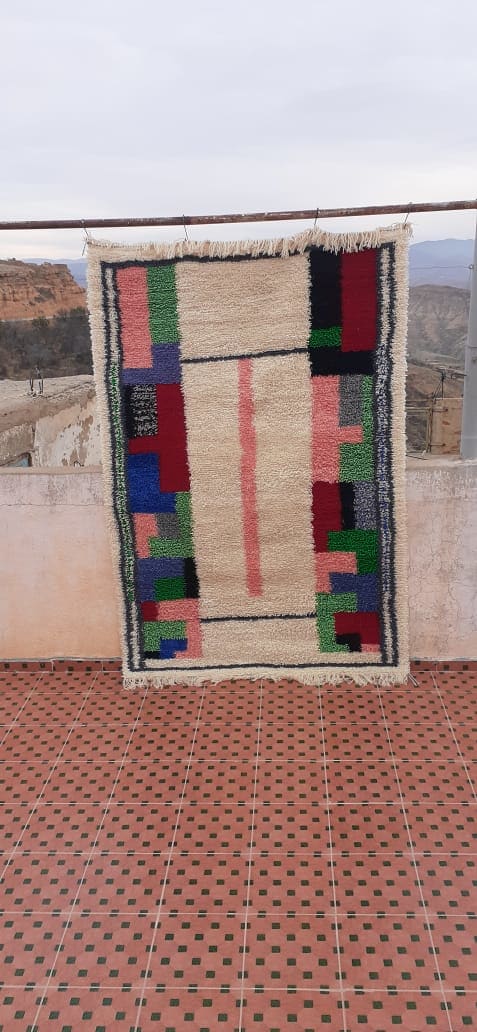This photograph captures an outdoor setting, likely a balcony with a white wall, overlooking a vast, rural landscape adorned with majestic, brown mountains or canyons. The floor of the balcony is a distinctive red tile interspersed with green and black checkered squares. Central to the composition is a handmade, woven rug suspended from a pole. The rug boasts a cream or beige background with a striking geometric design consisting of colorful shapes in red, black, pink, gray, blue, and green. Notably, there is a vertical pink stripe running down the center of the rug, flanked by thin black horizontal lines. The tapestry also features cream fringes at both the top and bottom. The intricate pattern, reminiscent of Tetris blocks, showcases a myriad of rectangles, T-shapes, and angles, contributing to its ornate appearance. This vivid arrangement juxtaposes beautifully with the natural backdrop, creating a scene that is both picturesque and rich in detail.